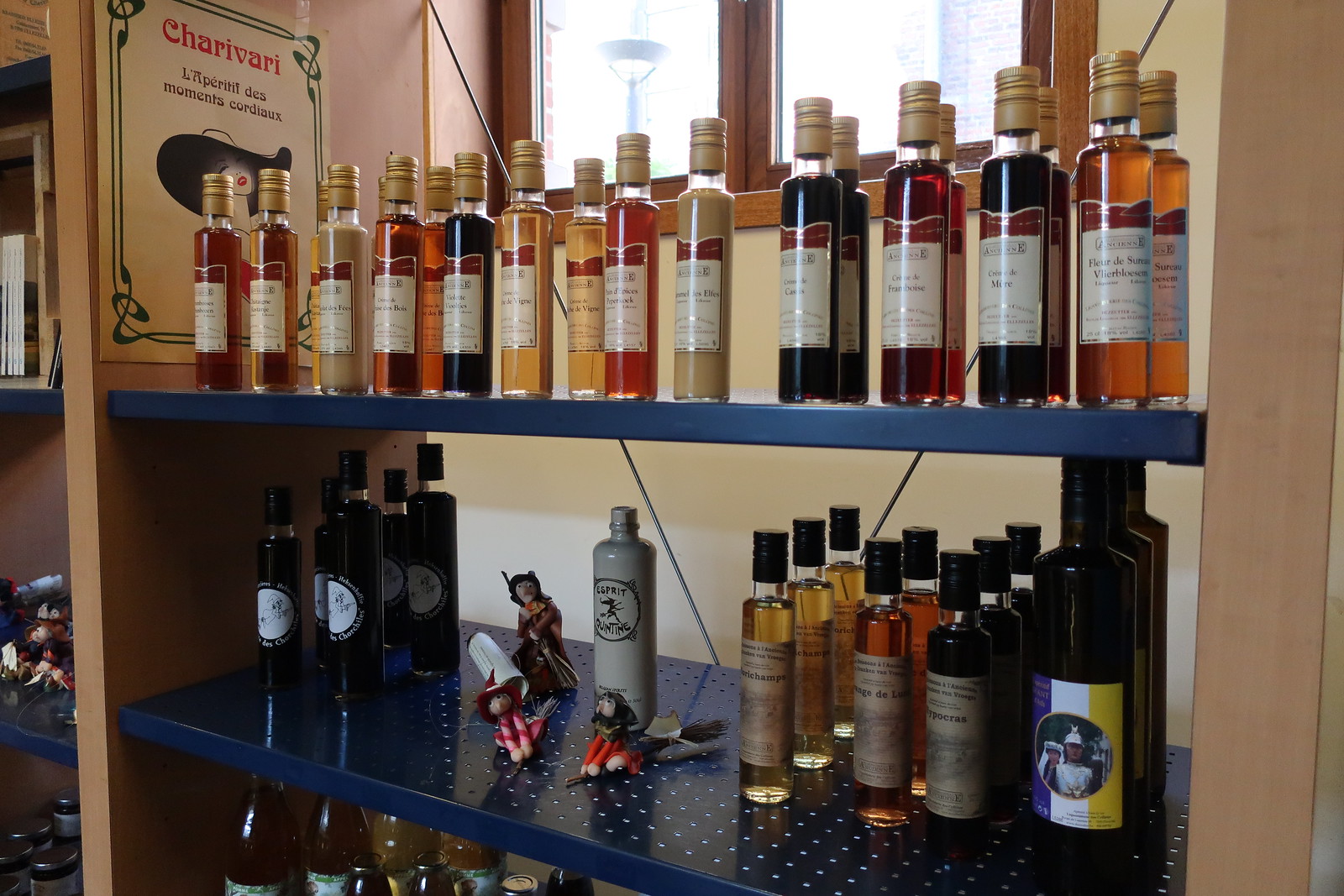The photograph captures a neatly organized set of blue metal shelves with perforations, featuring an extensive collection of artisanal vinegar bottles and decorative elements against a white wall. The shelves are structured with a tan-colored wooden frame and supported by an X-shaped cable at the back.

In the topmost shelf, a series of uniform glass vinegar bottles are prominently displayed. Each bottle features a clear body revealing a spectrum of liquids ranging from dark brown to amber, capped with plastic gold tops and adorned with uniform labels bearing white backgrounds and maroon headers. A variety of liquids, indicating different types of vinegar, fill these bottles, suggesting a sophisticated French origin through the elegant lettering on the labels.

To the left of the shelving unit, an off-white piece of paper with a green spiral border is taped to the frame. In red print, it announces "Charity Bardi" and below, in black, the French text "L'Aperitif de Moment Cordat," accompanied by an art deco image of a woman with a floppy hat and red lipstick.

On the middle shelf, a mix of vinegar bottles and three handcrafted figurines populate the space. The figurines appear to be witches in various flying poses with brooms. Situated among these figures is a non-transparent, white ceramic bottle featuring a label with the word "Esprit" and an image of a witch. Other bottles on this shelf have black caps and white labels, some containing golden yellow, brown, or black liquids.

Behind the middle shelf, visible through a window with a brown wooden frame, the outside streetlight and parts of a brick wall come into view.

On the lower visible shelf, additional vinegar bottles are observed, including dark-tinted bottles resembling wine bottles with intricate labels showcasing purple, white, and yellow vertical stripes. The labels feature images, possibly depicting a man with a white shirt and hat.

Overall, the detailed arrangement of shelves, variety of vinegar bottles, and quirky decorative accents contribute to a charming and meticulously curated display, suggesting an artisanal ambiance likely suited for a niche market or restaurant setting.